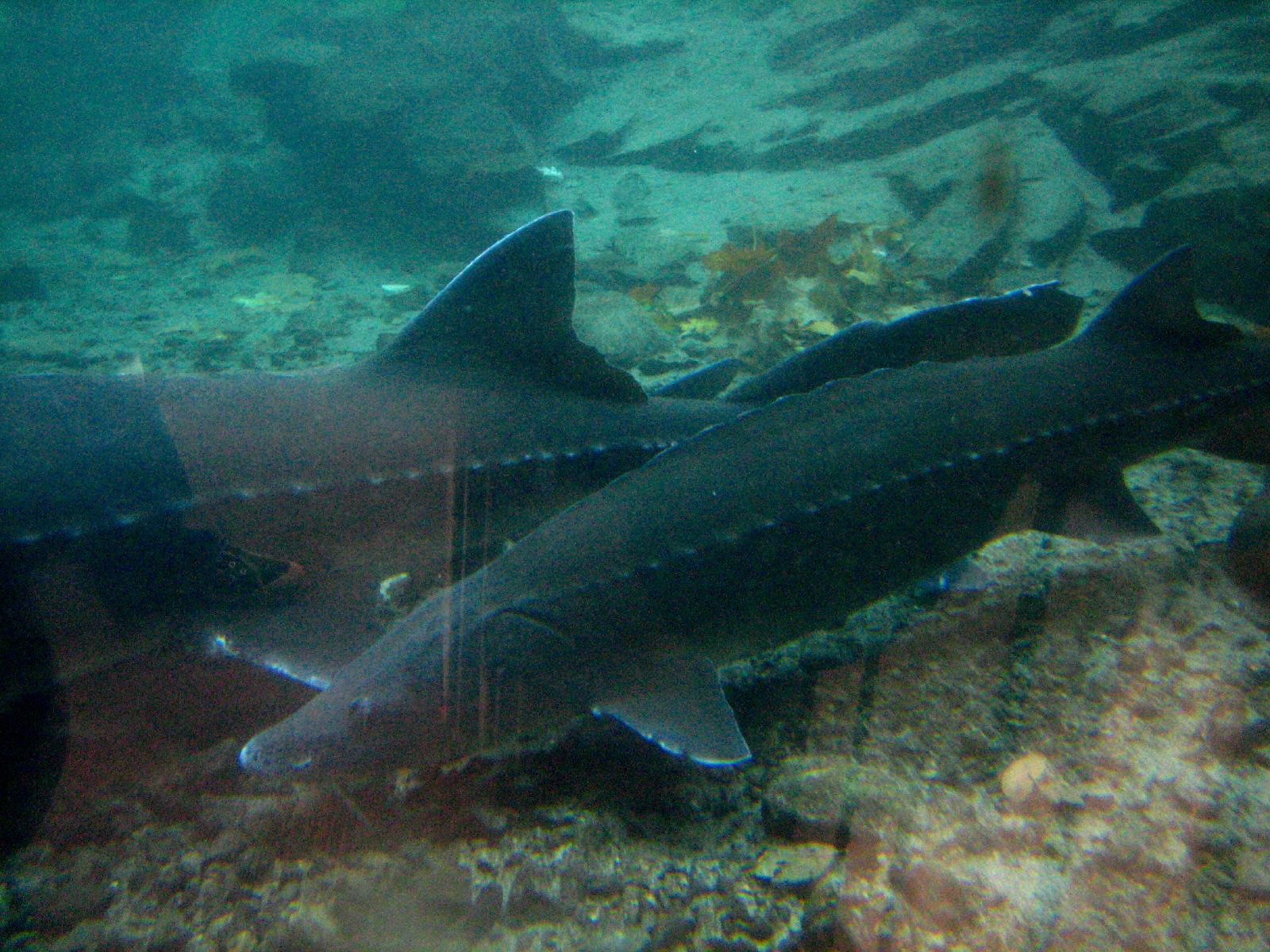The image depicts a scene set underwater, likely in an aquarium tank, viewed through a reflective glass surface. The main focus is on two large sharks swimming over a noticeably rocky and sediment-covered ground. One shark is significantly larger than the other, and both exhibit dark colors with some form of striping along their backs. The setting features a mix of colors, including gray, tan, brown, black, light blue, green, yellow, and orange, hinting at the diverse aquatic environment. The water is blue, and the scene reveals various smaller aquatic life forms in the background, along with elements resembling coral and gold flakes scattered around. The sharks are centrally positioned, with their prominent fins visible, emphasizing their dominance in the image as they swim forward together.